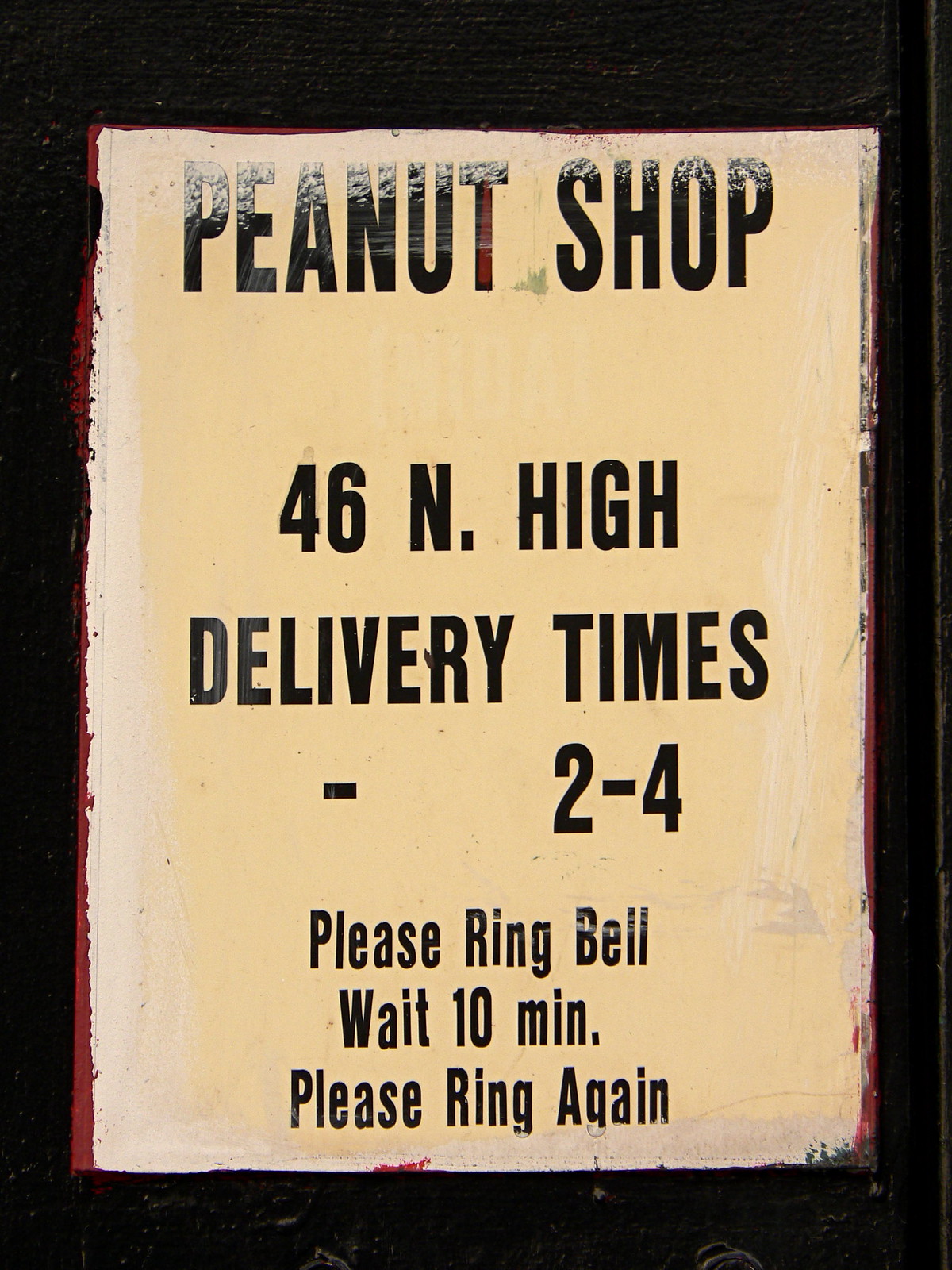The image captures a worn, yet stylish, rectangular sign that exemplifies the patina of aging. The sign is painted with a beige background and framed by a black border, peppered with hints of red paint suggesting layers of history. At the top, in striking black capital letters, the sign reads "PEANUT SHOP." Below, it lists the address as "46 N High," followed by "Delivery Times 2 to 4." Towards the bottom, it instructs, "Please ring bell, wait 10 min, please ring again," in smaller text. The sign's intricate layering and weathered look contribute to its charm. In the background, barely visible against the black wall, a small part of a doorknob peeks out, hinting at the presence of a door.